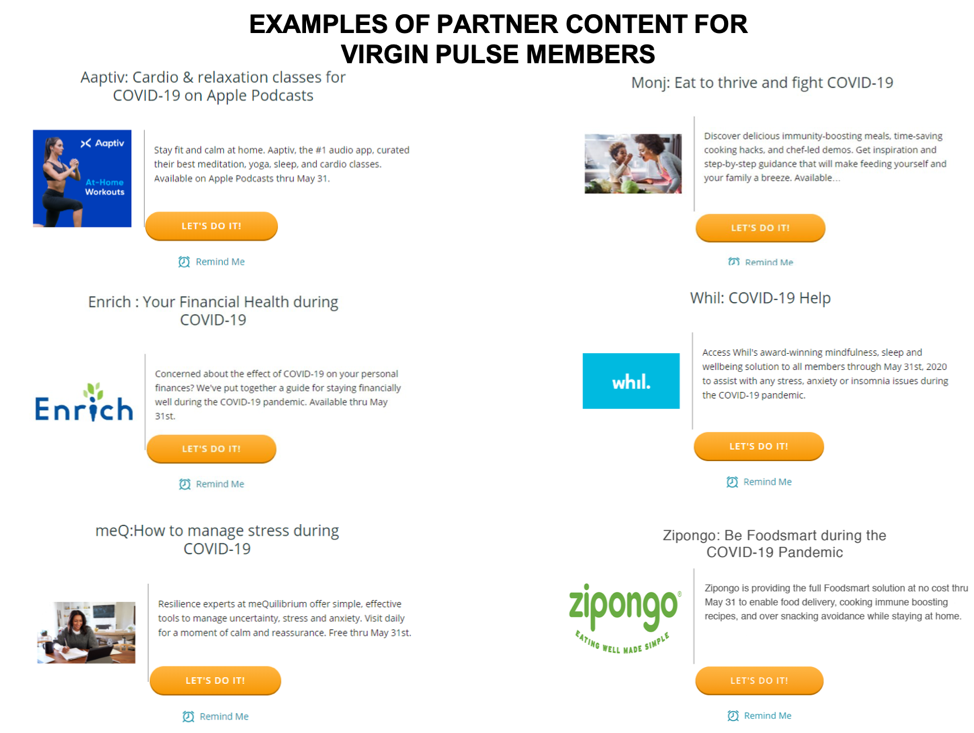The image features a white background with the title "Examples of Partner Content for Virgin Pulse Members" prominently displayed at the top. This title introduces various content resources designed to support individuals during the COVID-19 pandemic.

1. **First Section: Active Cardio and Relaxation Classes for COVID-19**  
   - **Image:** A blue square showing a woman exercising.  
   - **Text:** "Let's do it" in a yellow box with white print, accompanied by a smaller blue box saying "Remind me."  
   - **Platform:** Apple Podcast.

2. **Second Section: Enrich Your Financial Health During COVID-19**  
   - **Text:** Featured title "Enrich" in blue font, adorned with a green plant over the 'i' shaped like a person.  
   - **Buttons:** "Let's do it" in a yellow box and "Remind me" in a blue box.  

3. **Third Section: Me Q - How to Manage Stress During COVID-19**  
   - **Image:** A person sitting at a desk, presumably engaged in a stress-relief activity.  
   - **Buttons:** "Let's do it" in a yellow box and "Remind me" in a blue box.  

4. **Fourth Section: Monge eat to thrive and fight COVID-19**  
   - **Image:** A man and a little boy engaging in an activity.  
   - **Buttons:** "Let's do it" in a yellow box and "Remind me" in a blue box.  

5. **Fifth Section: Wow COVID-19 Help**  
   - **Image:** Small blue box with "Wow" written in white.  
   - **Buttons:** "Let's do it" in a yellow box and "Remind me" in a blue box.  

6. **Sixth Section: Zipongo - Be Food Smart During the COVID-19 Pandemic**  
   - **Text:** "Zipongo" in green, accompanied by the tagline "Eating well made simple."  
   - **Buttons:** "Let's do it" in a yellow box and "Remind me" in a blue box.  

Overall, the image effectively communicates a variety of supportive content, visually organized with titles, images, and actionable buttons to assist Virgin Pulse members during the challenging times of the COVID-19 pandemic.